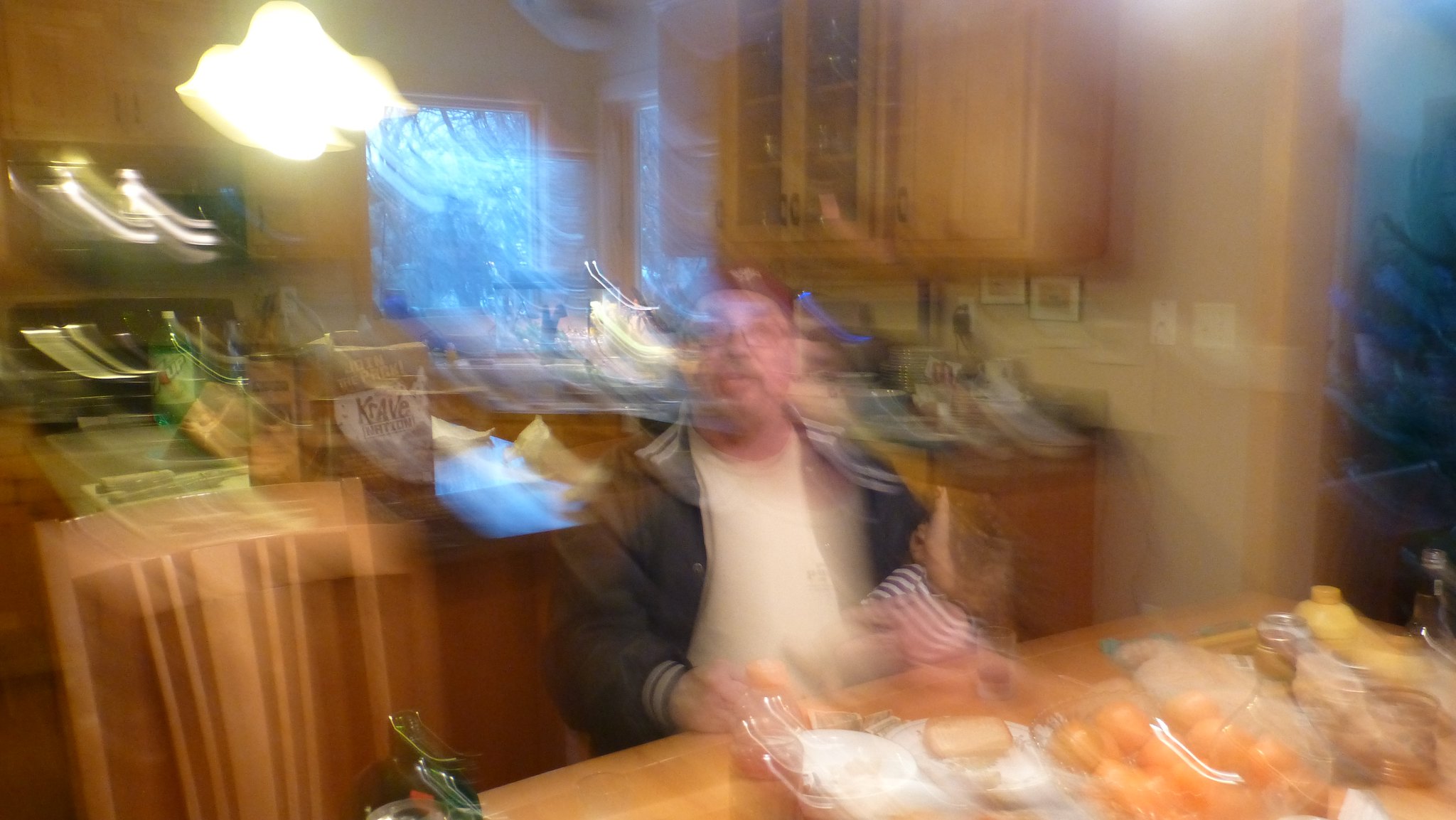In this candid, motion-blurred photograph taken inside a home, the focus is on an elderly man seated at a light brown wooden table within a cozy kitchen and dining room area. The man, wearing a dark blue jacket adorned with white stripes on the collar and sleeve ends, faces the camera with a direct yet unfocused gaze. His dark red hat, worn upside down, adds a touch of whimsical charm. Framed by prescription glasses, his small gray mustache hints at his advanced age. The kitchen backdrop features a central island cluttered with various food items and a soda, hinting at recent activity. A chandelier light fixture hangs above, illuminating light brown cupboards in the upper right corner and a countertop that stretches into the room's corner. A window near the center-left side brings in natural light, rounding out this intimate glimpse into a lived-in home setting.